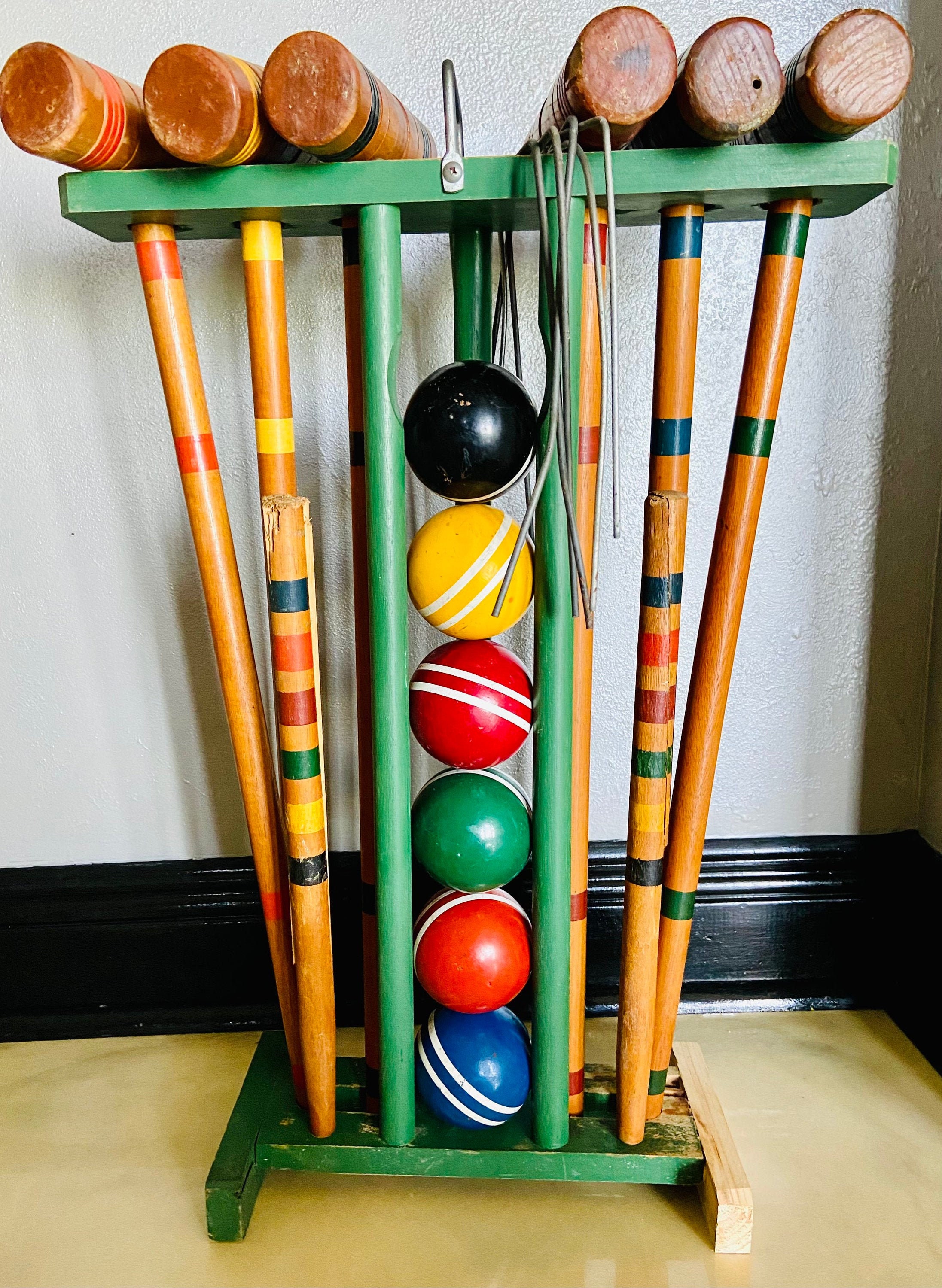In the photograph, a green wooden croquet set holder is displayed prominently, with a silver handle affixed at its center. Positioned inside the holder are six wooden mallets, each brown in color and adorned with various colored tapes or stripes, including yellow, blue, red, and green. These mallets are symmetrically arranged, with three on each side. Down the center of the holder is a compartment housing six croquet balls, each marked by two white horizontal stripes. The balls are stacked in the following order from top to bottom: black, yellow, red, green, orange, and blue. The background features a gray wall with a black baseboard and a light brown floor, adding contrast to the scene. Some parts of the green paint on the holder are faded, revealing the wood beneath, and one section of the wood appears newer and unpainted.